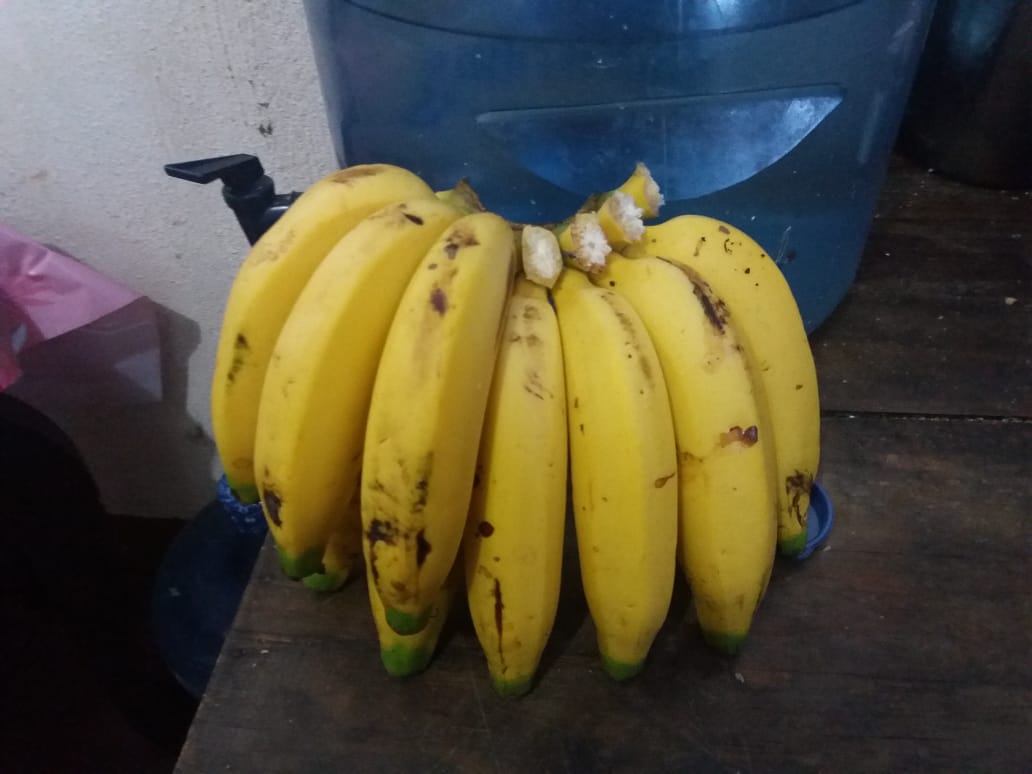In a dimly lit indoor setting, this color photograph captures a rustic scene centered around a bunch of ripe bananas lying on a dark brown wooden table. The yellow bananas, speckled with brown spots and with slightly green tips, are arranged with their bottoms facing up. Four bananas have been removed from the bunch, leaving behind cleanly cut stems. Peeking from beneath the bananas is a blue cap. In the background to the right, a large blue plastic water jug, topped with a cap, dominates the scene. To the left, a somewhat shabby white wall shows signs of wear with visible spots and possibly a fragment of a pink disposable tablecloth clinging to it. The overall atmosphere is one of casual neglect, with details like a small piece of paper on another nearby table and the edge of an unseen object forming part of the composition.